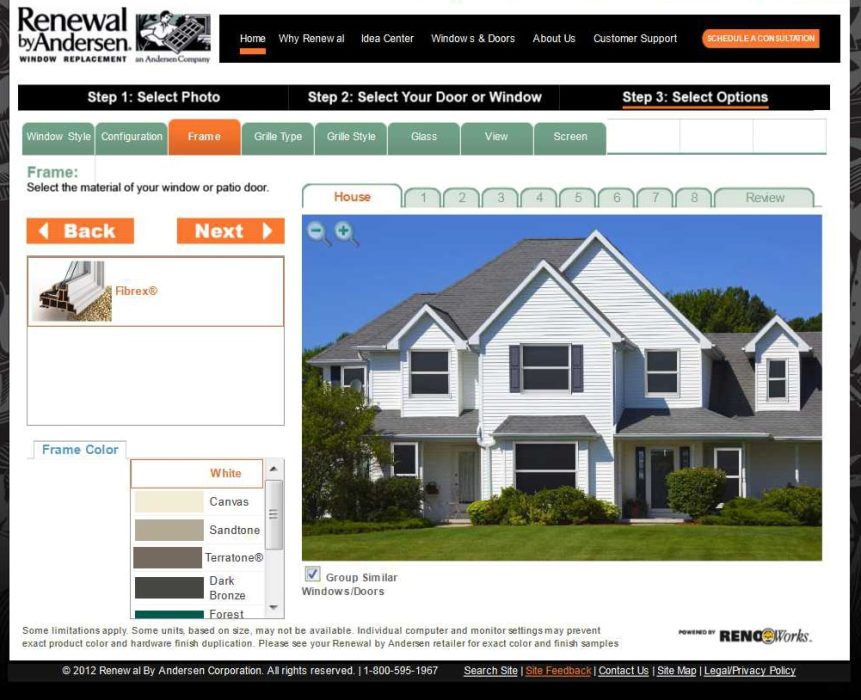This image appears to be a screenshot from a website dedicated to window replacement services, specifically from Renewal by Andersen. The overall shape of the photo is square with a predominantly white background. In the upper left corner, the logo "Renewal by Andersen" is displayed in black font, accompanied by the phrase "Window Replacement" and a cartoon image of a man carrying a window.

To the right, there's a long, rectangular black navigation bar with white text. The options listed in the navigation bar include: Home, Why Renewal, Idea Center, Windows and Doors, About Us, and Customer Support. There's also an orange oval button that appears to be a "Schedule a Consultation" option, though the text is partly obscured.

Below the navigation bar, the "Home" tab is highlighted with an orange border, indicating it is currently selected. The main content area beneath this contains three instructional columns: 
1. Select Photo
2. Select Your Door/Window
3. Select Options (underlined in orange).

There are multiple green bubbles beneath these instructions, each representing a different customization option: 
- Window Style
- Configuration
- Frame (currently selected and highlighted in orange)
- Grill Type
- Grill Style
- Glass View
- Screen

At the bottom of the image, there is a picture of a house which seems to serve as an interactive model. Users can customize this house to visualize different window options and frame colors.

The website seems designed to guide users through the process of selecting and customizing their new windows step by step, providing visual aids and interactive elements to help with their decisions.